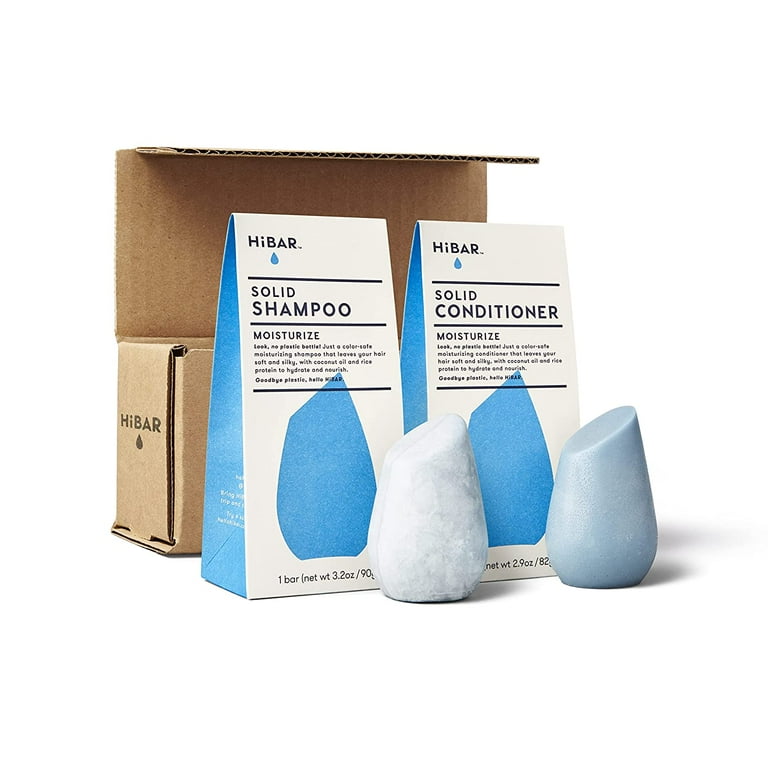The image showcases two related hair care products from the brand Hi-Bar: a solid shampoo and a solid conditioner. Both products are solid bars instead of liquid formulations. The shampoo is white, while the conditioner is a pale blue. Each bar is uniquely shaped like a droplet, with a slight slant on the top, resembling the slant of a lipstick. The pair of bars is positioned in front of their respective packaging boxes, which are white with blue accents and black text. The packaging prominently displays the Hi-Bar branding and the words "Solid Shampoo Moisturize" and "Solid Conditioner Moisturize." These items were originally shipped in a brown cardboard box, which is seen open in the background of the image. This cardboard box also bears the Hi-Bar logo.